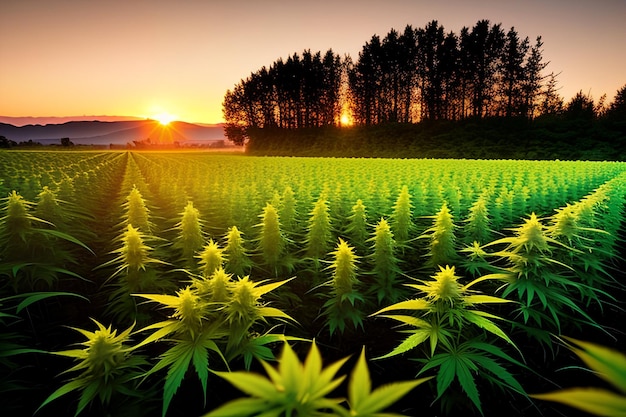This digitalized painting captures an expansive, verdant field filled with acres of green plants that resemble marijuana, arranged in orderly rows that span miles. The plants are characterized by their oval-like, pointy green leaves and spiky, cone-shaped clusters. Dominating the lower half of the image, the field appears lush and herbaceous. As the scene unfolds, the striking background reveals a picturesque, low-lying mountain with grayish-blue tones, accompanied by huge, imposing trees with thin trunks and bushy tops silhouetted against a vividly colorful sunset sky. The heavens are painted in shades of red-pink, purple, and orange, with the golden glow of the setting sun illuminating the tops of the plants and casting a serene, magical light over the landscape. To the far left, the sun dips behind the mountains, appearing to kiss the horizon, while faint outlines of possible buildings or homes nestled at the base of the hills hint at a tranquil, pastoral life.